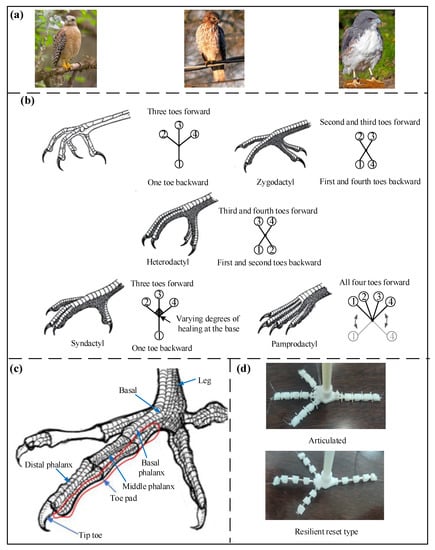The image is a detailed drawing displaying various birds, identified as falcons and eagles, along with their distinct claws. The photograph section is labeled with a lowercase 'a,' featuring wild birds perched on trees, affirming their non-domesticated nature. The top section showcases three bird images followed by close-ups of their claws below. The specified labels on the claws include "toes forward" and "one toe back, three toes forward," highlighting the differences in their talon structure. The colors appearing in the image are a mix of green, light brown, light red, gray, white, and black. This composition emphasizes the unique physical adaptations of the birds for catching and carrying prey.